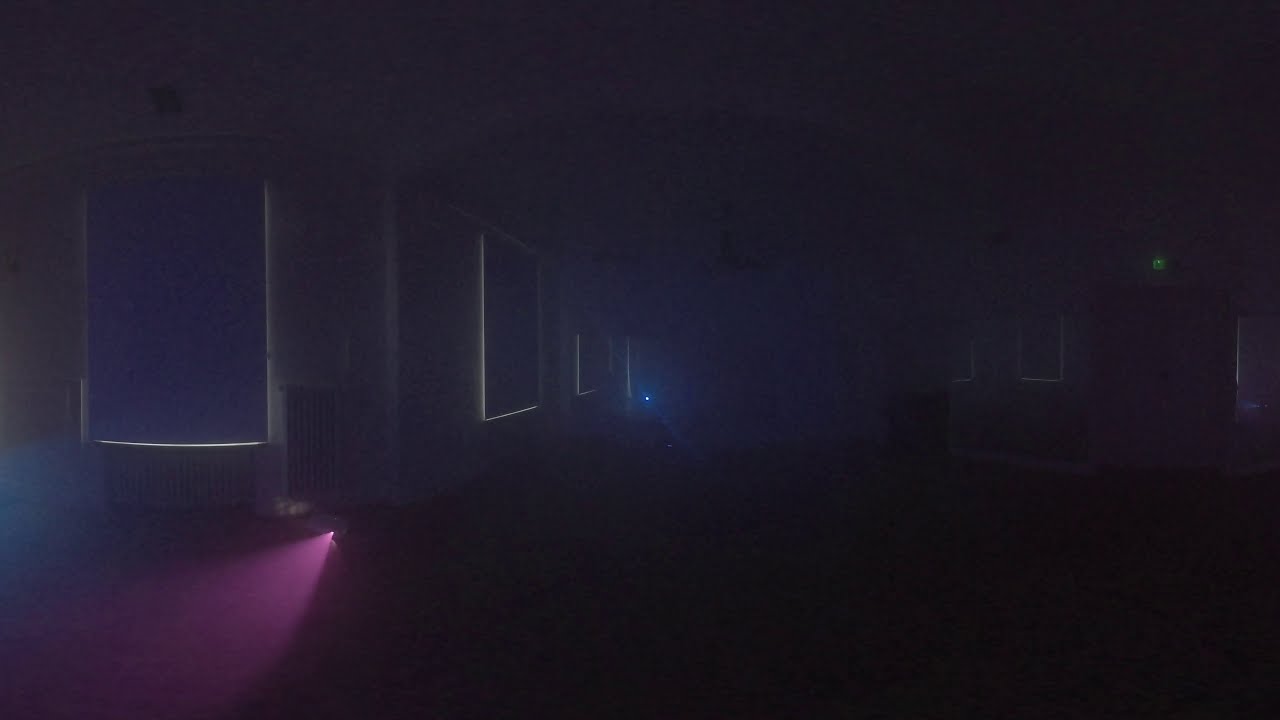In this image, we see a dimly lit, predominantly dark blue or navy room with a curved wall. The wall features windows at the far end, covered with curtains, allowing a small amount of sunlight to seep through the edges and bottom. The floor appears to be red or magenta and seems slightly foggy or smoky, especially near the bottom left corner where a bright pink light shines. This light originates from a single point and spreads out in a cone shape, illuminating part of the floor. Just left of the center, there's a blue orb-like light source, adding to the room's ethereal ambiance. There is also a green light, likely an exit sign, above a door frame on the right side, suggesting an emergency exit.